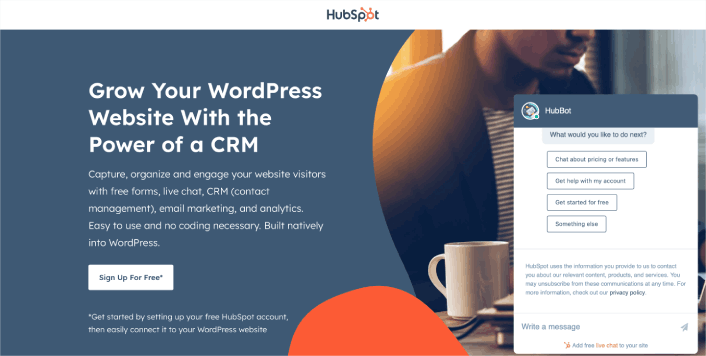The image features a promotional web page designed in a bluish-gray color palette. Dominating the white space is the prominent HubSpot logo, characterized by the word "HubSpot" where the letter 'O' is stylized with radiating spikes. The central message in bold white text reads, "Grow your WordPress website with the power of a CRM." Beneath this, in a lighter shade of white, additional details are provided: "Capture, organize, and engage your website visitors with free forms, live chat, CRM (contact management), email marketing, and analytics. Easy to use and no coding necessary. Built into WordPress."

A white call-to-action rectangle near the bottom of the web page invites users to "Sign up for free*." An asterisk leads to a smaller text explaining, "Get started by setting up your free HubSpot account, then easily connect it to your WordPress website."

In the background, there is a partial image of a man, featuring only his neck, chest area, and a coffee cup. An orange half-moon shape is visible at the bottom of the image, adding a touch of vibrant color. To the right, a superimposed white rectangle provides further information about the HubSpot offering.